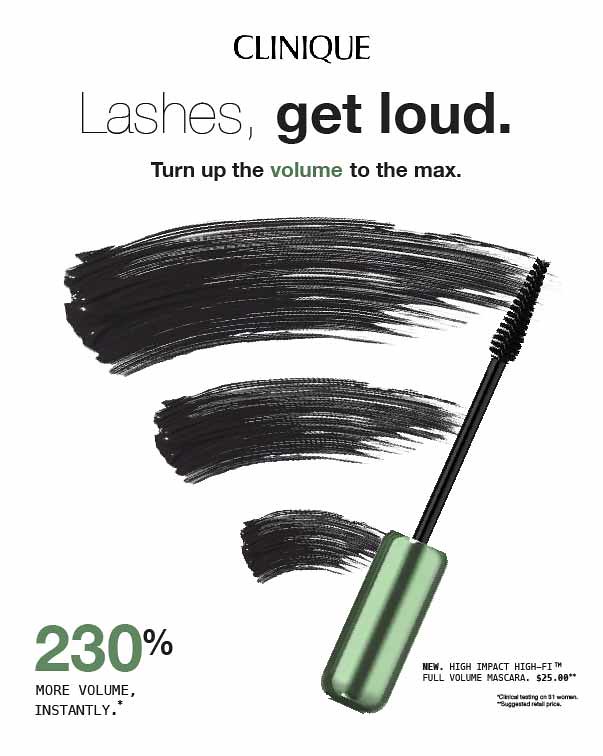Promotional image for Clinique's new High Impact Hi-Fi Full Volume Mascara, priced at $25. The top of the image prominently features the brand name "CLINIQUE" in black text. Below it reads, "Lashes Get Loud. Turn up the volume to the max," emphasizing dramatic lash enhancement. Centered on a white background is a mascara stick with a green cap and a black brush, creating three bold black streaks that progressively diminish in size, resembling marker lines. The bottom left corner displays "230% More Volume Instantly" with "230%" in green text. In the bottom right corner, the ad specifies, "New High Impact Hi-Fi Full Volume Mascara $25" in black text. The overall design draws attention to the product's promise of significantly enhancing lash volume.